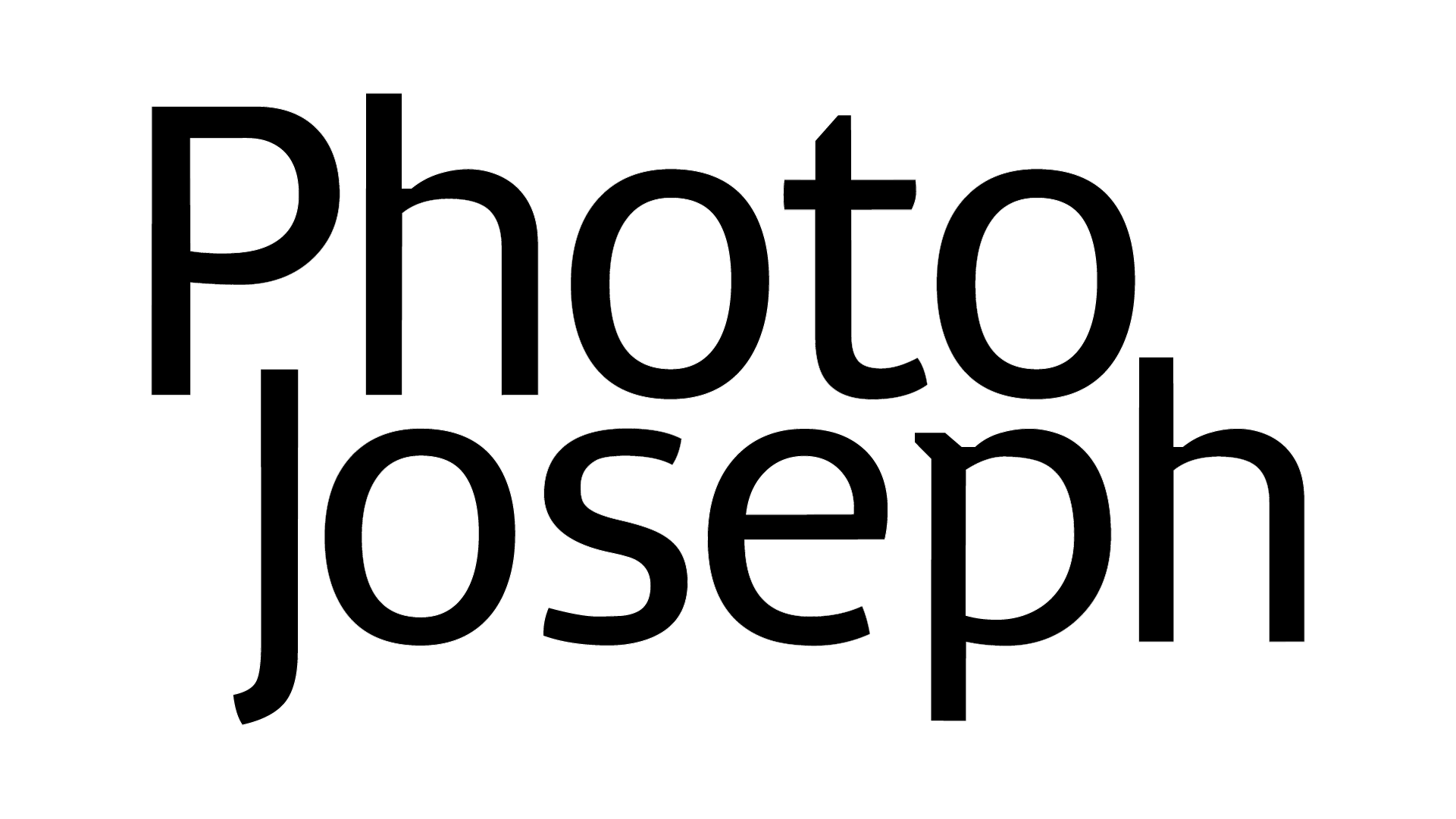The image features large black text on a clean white background, with no additional elements or colors. The text spans two lines, each rendered in a substantial, approximately 16-point font with a medium weight. The first line reads "Photo," starting with an uppercase 'P' followed by lowercase 'h', 'o', 't', and 'o'. The second line reads "Joseph," beginning with an uppercase 'J' followed by lowercase 'o', 's', 'e', 'p', 'h'. The font used is not Times New Roman but a more contemporary, computer-friendly style. The text appears centered on the page, giving the impression that "PhotoJoseph" is potentially a company name. The overall minimalistic design suggests it could be utilized on a website or business cards.